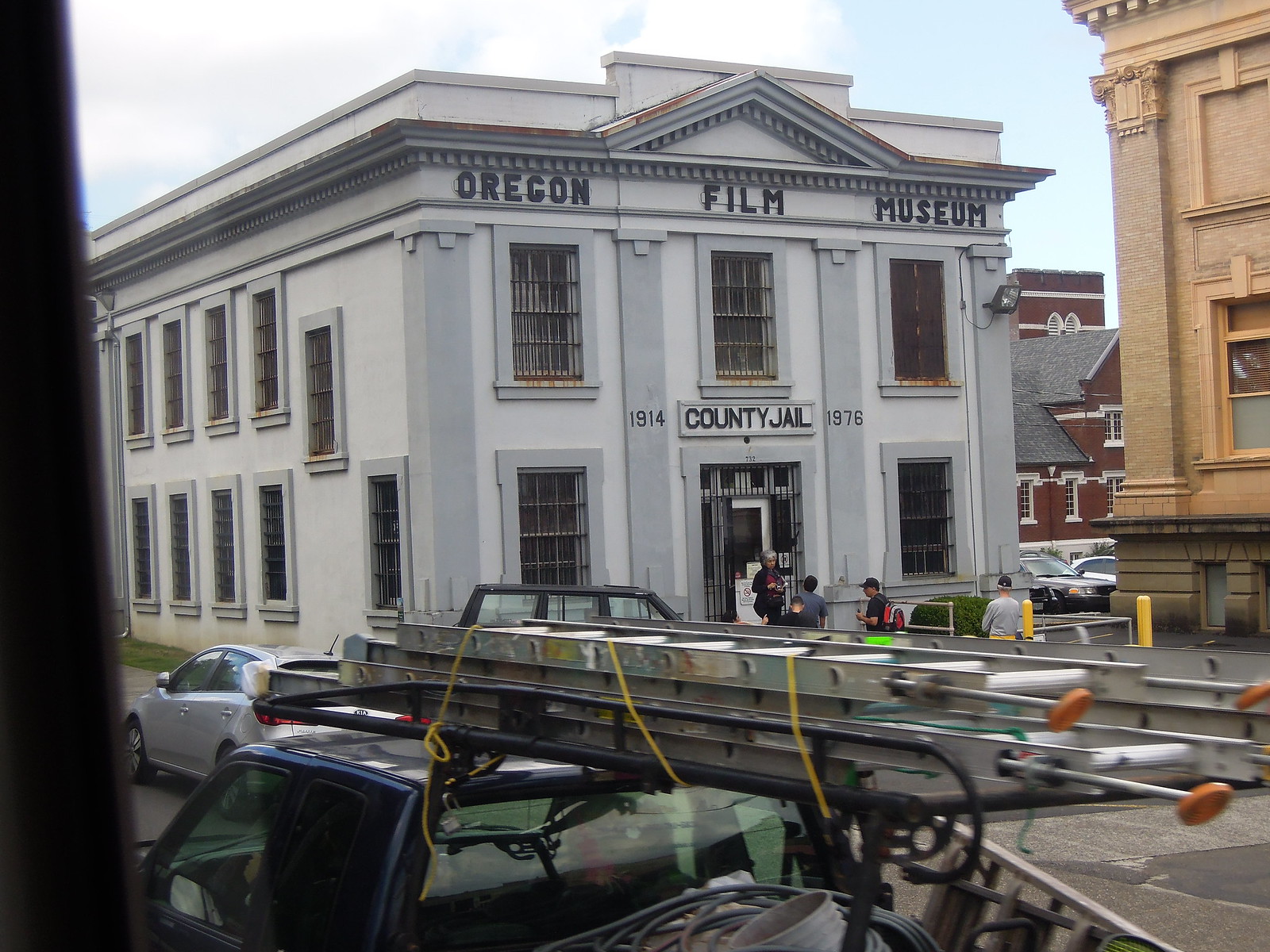The photograph captures a detailed outdoor scene of an old gray stone building prominently labeled "Oregon Film Museum" at its top. This two-story structure, also marked as the "County Jail 1914 - 1976," features a front facade with three barred windows on the upper floor and two on the ground level flanking a central doorway. To the left, the long side wall of the building exhibits multiple barred windows, totaling ten.

A blue pickup truck, equipped with silver ladders on its roof and various hoses and equipment in its bed, is positioned prominently in the foreground facing the museum. Nearby, another car, a Kia, is visible on the street. The scene also includes four men of various ages standing outside the entrance, engaging with a woman who stands at the doorway, possibly exiting or conversing with them.

In the background, on the left, a red brick building with white window trims and a gray roof, reminiscent of a church due to its steep slate roofing and tower, complements the historic character of the area. On the right, partially visible, is another structure featuring a gray masonry brick foundation and tan columns. The sky is brightly blue with clouds gathering on the left side, providing a crisp, clear contrast to the historic, stone-faced architecture below. This emphasizes the rich, storied past of this Oregon locale.